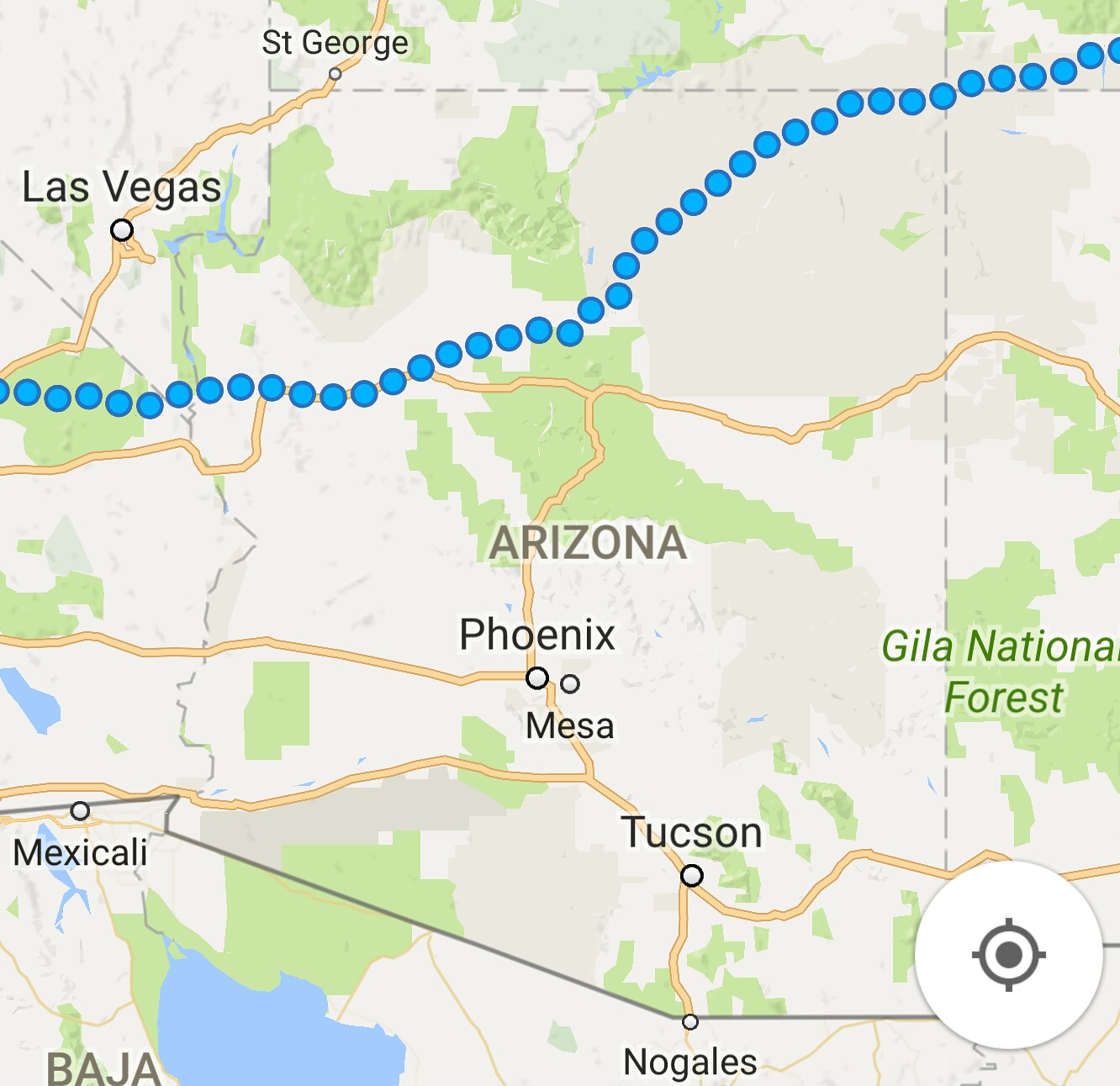The image features a detailed map centered on the state of Arizona, prominently labeled in the middle. Major Arizona cities like Phoenix, Mesa, and Tucson are clearly marked. The map also highlights key locations in neighboring areas: Las Vegas sits in the top left corner, while St. George, Utah lies along the same highway intersection. Mexico is visible to the south, with Nogales at the border and Mexicali positioned near the California and Baja California borders. The highways across Arizona are depicted, including a notable stretch of I-10 running from Phoenix to Tucson, though none are labeled. Additional geographical features include the Gila National Forest on the right, blue dots forming a line across the top of the map, and scattered green spots within the predominantly beige-colored region. At the map's bottom right, there is a white dot with a bullseye pattern.